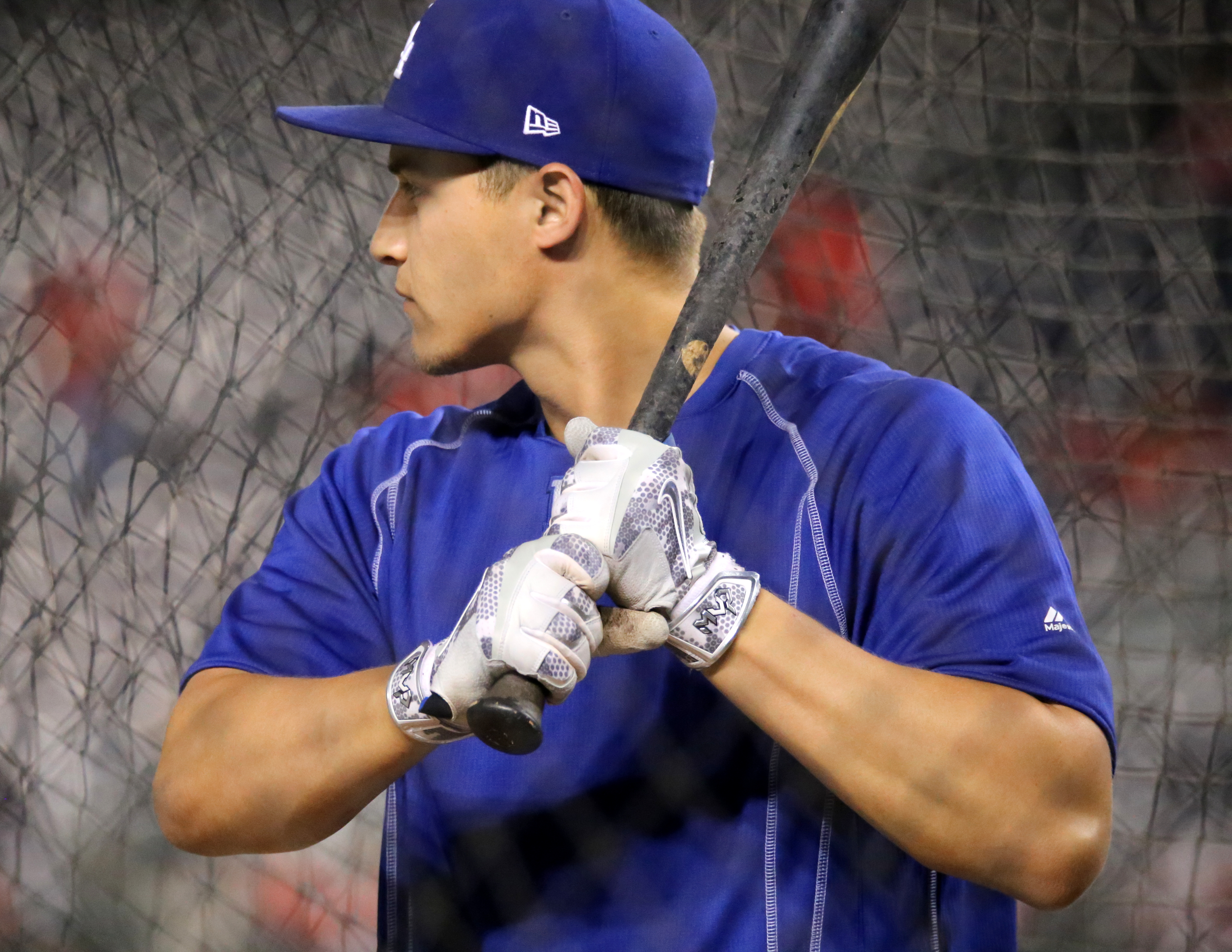The image showcases a baseball player during batting practice. He is wearing a blue jersey with white piping and a white logo that says "Major..." in a triangle near his elbow. The jersey is plain without any numbers. He also has on a blue New Era baseball cap featuring a white "N" logo, and short brown hair peeks out from underneath. The player's hands are clad in white gloves with blue patterns as he grips a black bat with traces of orange and pine tar, indicating usage. The bat is positioned over his shoulder, and he is poised to swing with his left hand. The background is blurred, revealing a black netting and indistinct red blobs, likely equipment or distant objects. The image captures his torso and side profile, presenting a dynamic and focused moment.